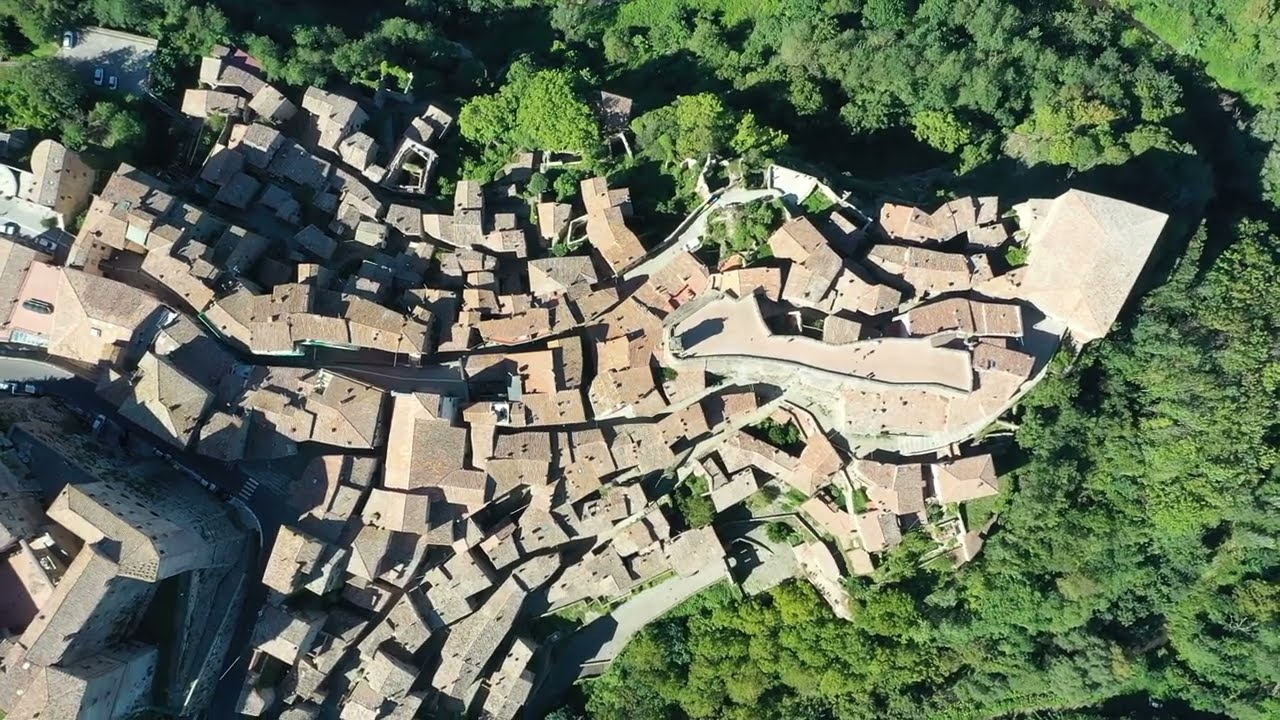This aerial photograph captures a picturesque hillside neighborhood with peach and tan-colored rooftops, nestled closely within groves of bright green trees. The densely packed homes are oriented around a winding one-lane road that encircles the area, giving the impression of a historic European village, possibly in Tuscany. The landscape gradually slopes from higher elevations on the right to a lower central valley, then rises again towards the left, creating a dynamic and tiered layout. In the center-right of the image, there's an open town square, where small figures, likely residents, can be seen walking about, suggesting a communal focal point. The neighborhood is interspersed with some commercial and apartment buildings and is bordered by lush trees and possibly a body of water, enhancing its secluded and charming appeal.